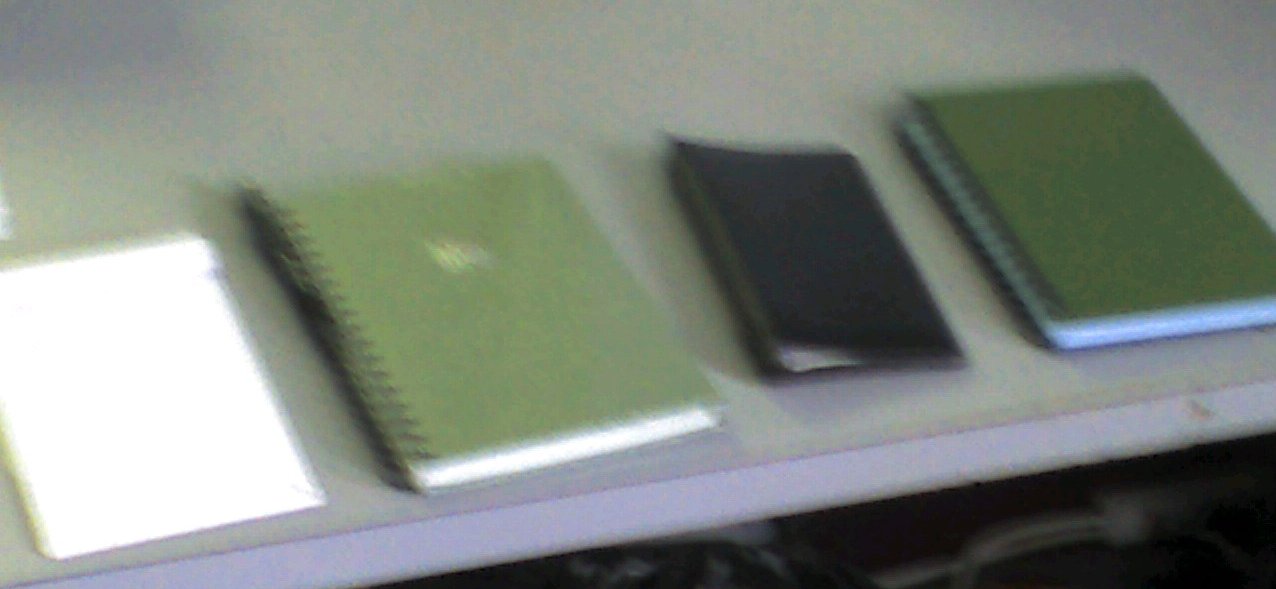This photograph, though out of focus, captures four different types of organizers spread out on a gray shelf or desk. From left to right, there is a bright white, tablet-style planner or memo pad. Next to it is a green spiral-bound notebook with a hint of gold, featuring white pages and a touch of pink in the middle. On its right is a small black notebook, which also appears to be spiral-bound with white paper peeking out along its edge. Lastly, on the far right, is another green notebook with a white paper spine. Despite the lack of clarity, the image distinctly displays this variety of organizing tools.